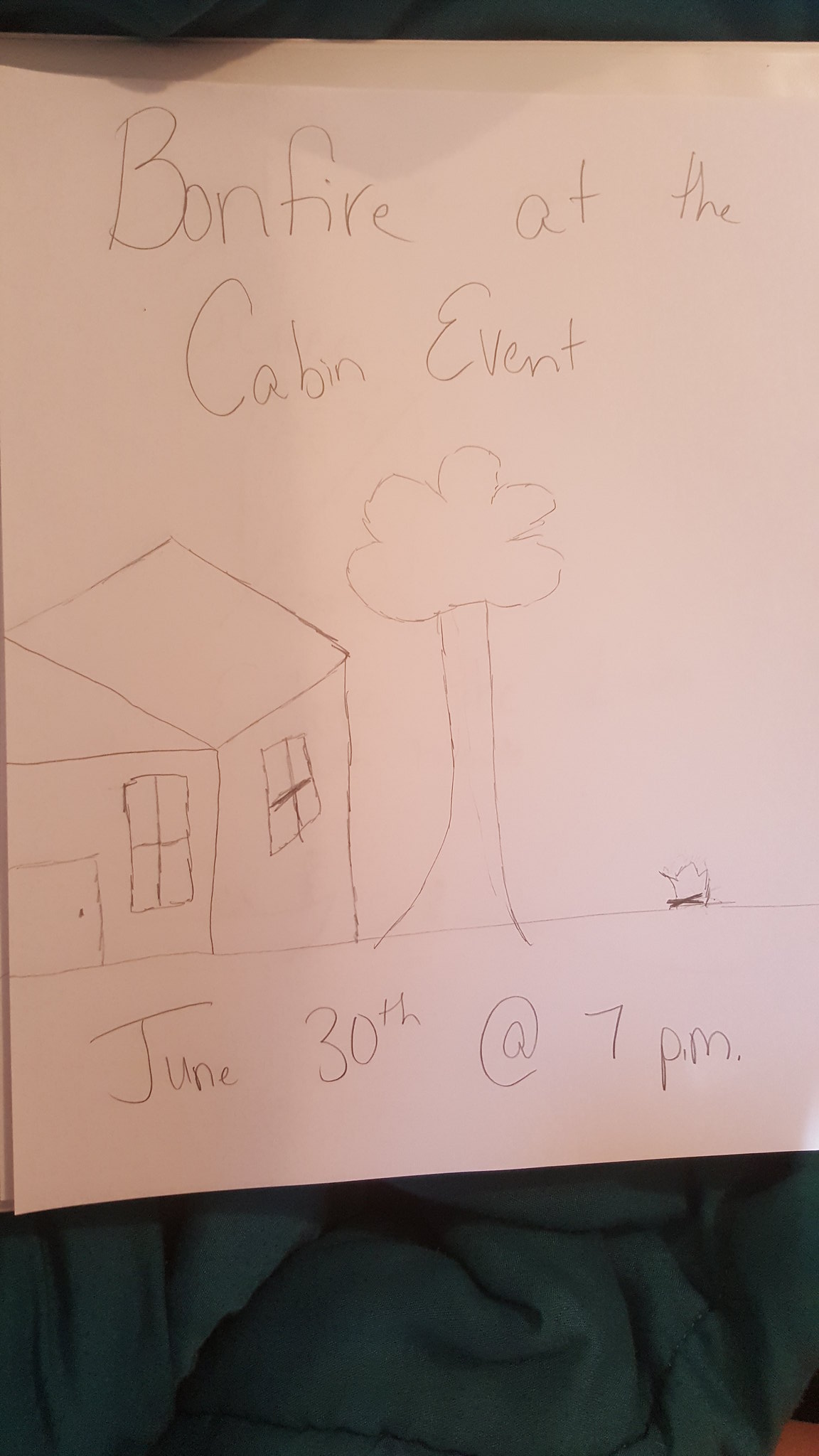This is a photograph of a simplistic pencil drawing on a sheet of paper, announcing a "Bonfire at the Cabin Event." The drawing features a rudimentary depiction of a house on the left, a tree in the middle, and a small bonfire represented by a squiggle on the right side of the paper. The event details, "June 30th at 7 p.m.," are written at the bottom. The paper, which has a different textured top likely for tearing off, is placed on a dark green cloth or mattress fabric. The lighting in the photograph is poor, and part of a person's clothing is visible at the edge of the image. The drawing appears hastily done, possibly by a child, while the lettering seems more mature.